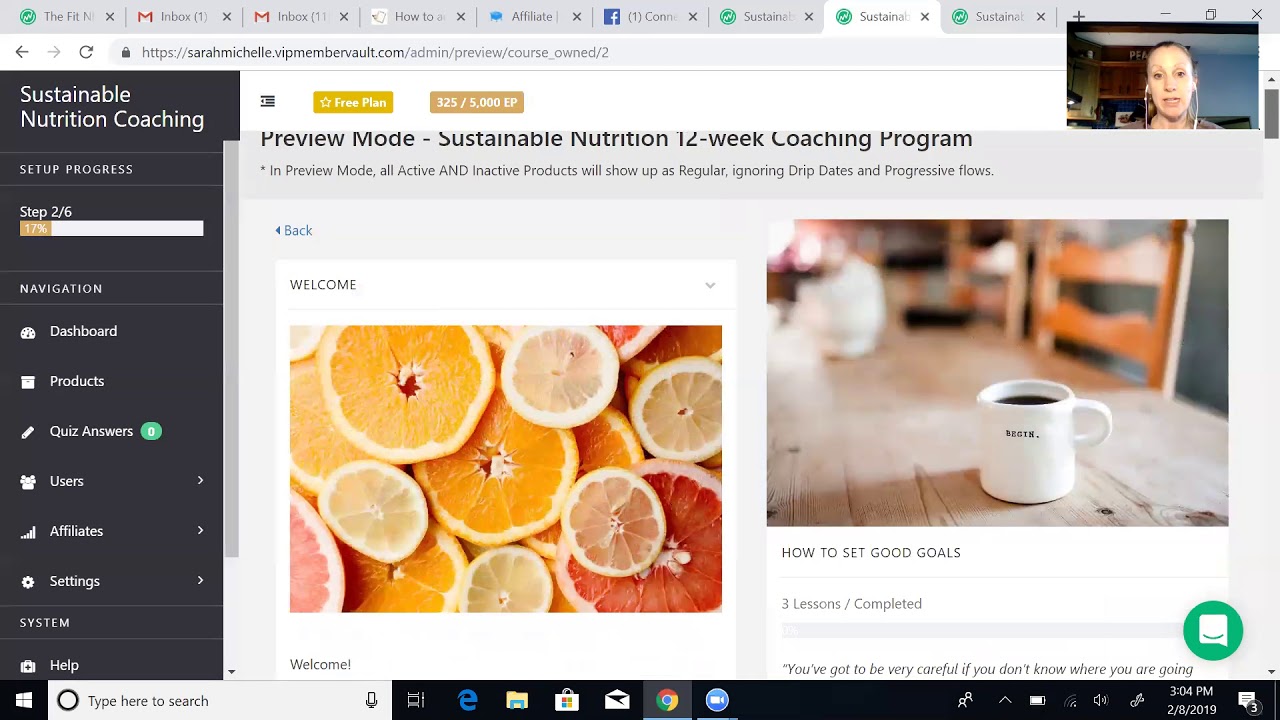The computer screen in the image has multiple tabs open at the top, including "The Fit," two inbox tabs, "How To," "Affiliate," Facebook, and three tabs labeled "Sustainable." In the upper right corner, there's a small pop-up showing a woman with headphones on, standing in a kitchen with a blue wall behind her, indicating she is on camera. The URL bar at the top reads "sarahmichelle.vipmembervault.com," suggesting the website is related to nutritional coaching.

On the left side of the screen, there is a black sidebar displaying "Sustainable Nutrition Coaching." Below that, it shows "Setup Progress" at 17%, referring to "Step 206." The navigation menu includes options like Dashboard, Products, Quiz Answers, Users, Affiliates, and Settings.

The main content area is in "Preview Mode" and features the "Sustainable Nutrition 12 Week Coaching Program." Below this title is an image of orange slices with a "Welcome" message above it. To the right, there is another image of a coffee cup on a table with the text "How to Set Good Goals."

Overall, the screen provides an overview of a nutritional coaching program interface with various educational and setup components visible.